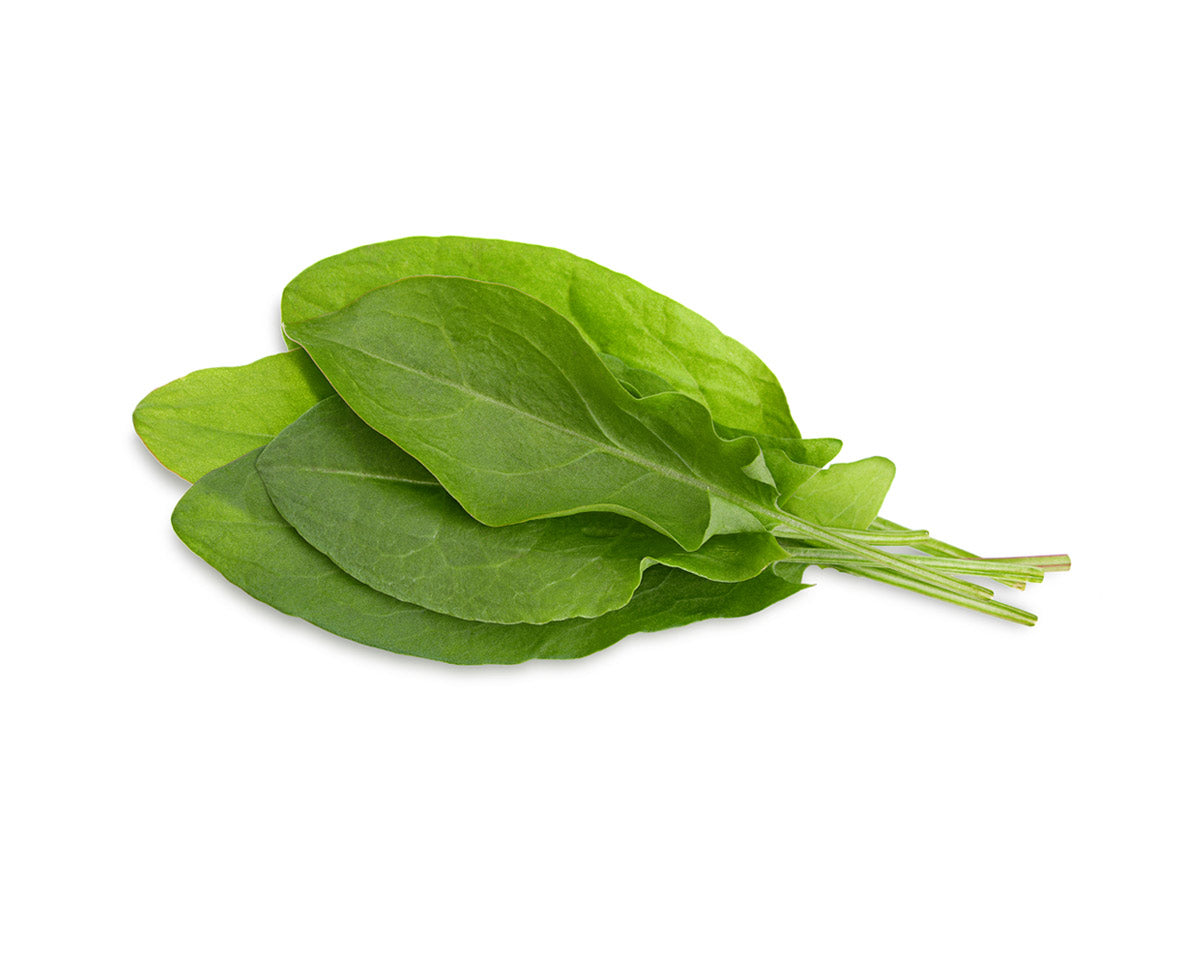This image captures a close-up of five oblong, leafy greens, meticulously stacked on a clean, white background. Each leaf, possibly basil, arugula, or spinach, lies with its stem extending to the right while the foliage fans out to the left. The arrangement features a mix of leaf sizes and shades of green, with the bottom leaf being the longest and lightest in color, and the top leaf shorter and darker. The veins are faint but visible, showcasing the intricate details of the leaves. Lighting is soft, enhancing the freshness and texture of the greens, suggesting it might be a stock image or possibly used in a culinary blog post.